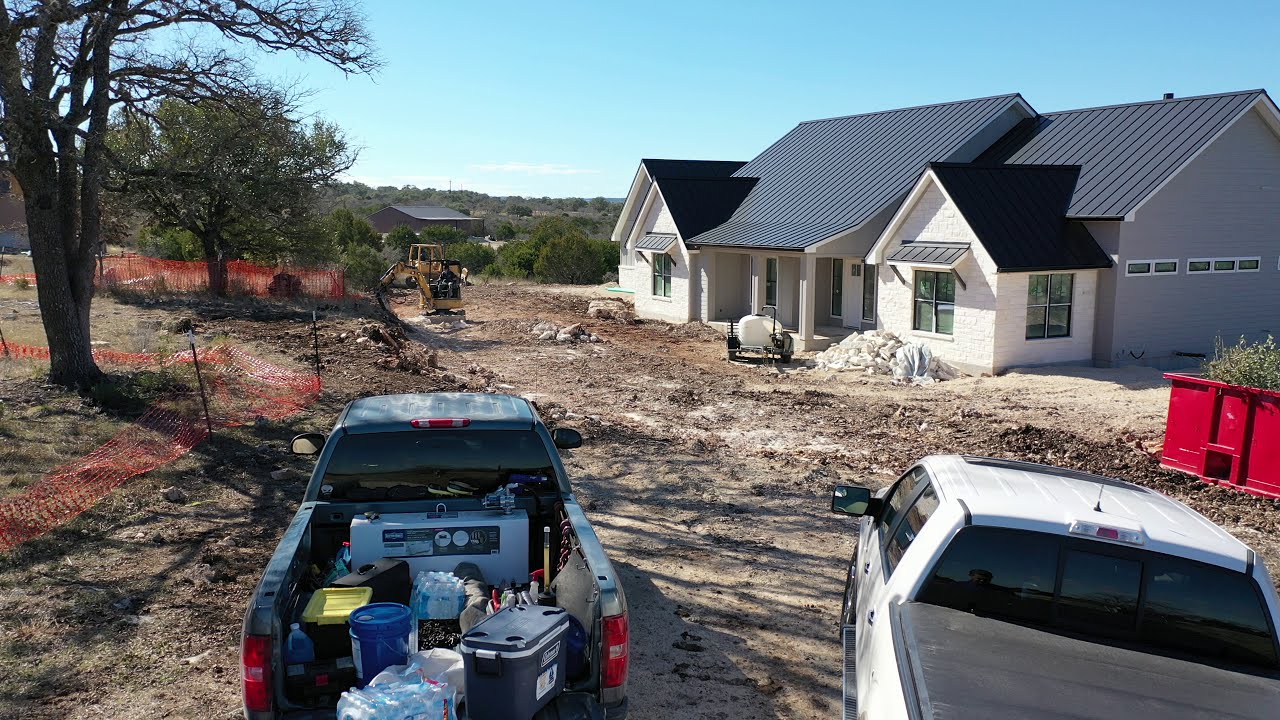This detailed photograph captures a house under construction from what appears to be an elevated perspective. The house features a distinctive conical roof painted dark blue and a mix of white and light gray external walls. On the right side of the house, horizontally oriented windows add to its modern aesthetic. The house's entry is recessed, framed by protruding wings.

In the foreground of the image, the ground is rough, covered in sand, soil, and rocks — evidence of ongoing construction. Notably, there are several pieces of construction equipment, including a skid steer excavator with its bucket digging into the earth, indicative of active excavation work.

Parked in the middle of the frame are two mini trucks: a white one with a tonneau cover and sliding back glass and a blue or hunter green one filled with various contractor supplies. The blue truck's bed contains items such as a gray Coleman cooler with cup holders, a blue five-gallon paint bucket, a white rectangular box, and a dark-colored bucket with a yellow lid.

Adding to the dynamic scene are some trees on the left side, shielded with red-colored nets, and additional building structures can be glimpsed further away. The sky above is clear and blue, providing a serene backdrop to the bustling construction activity below.